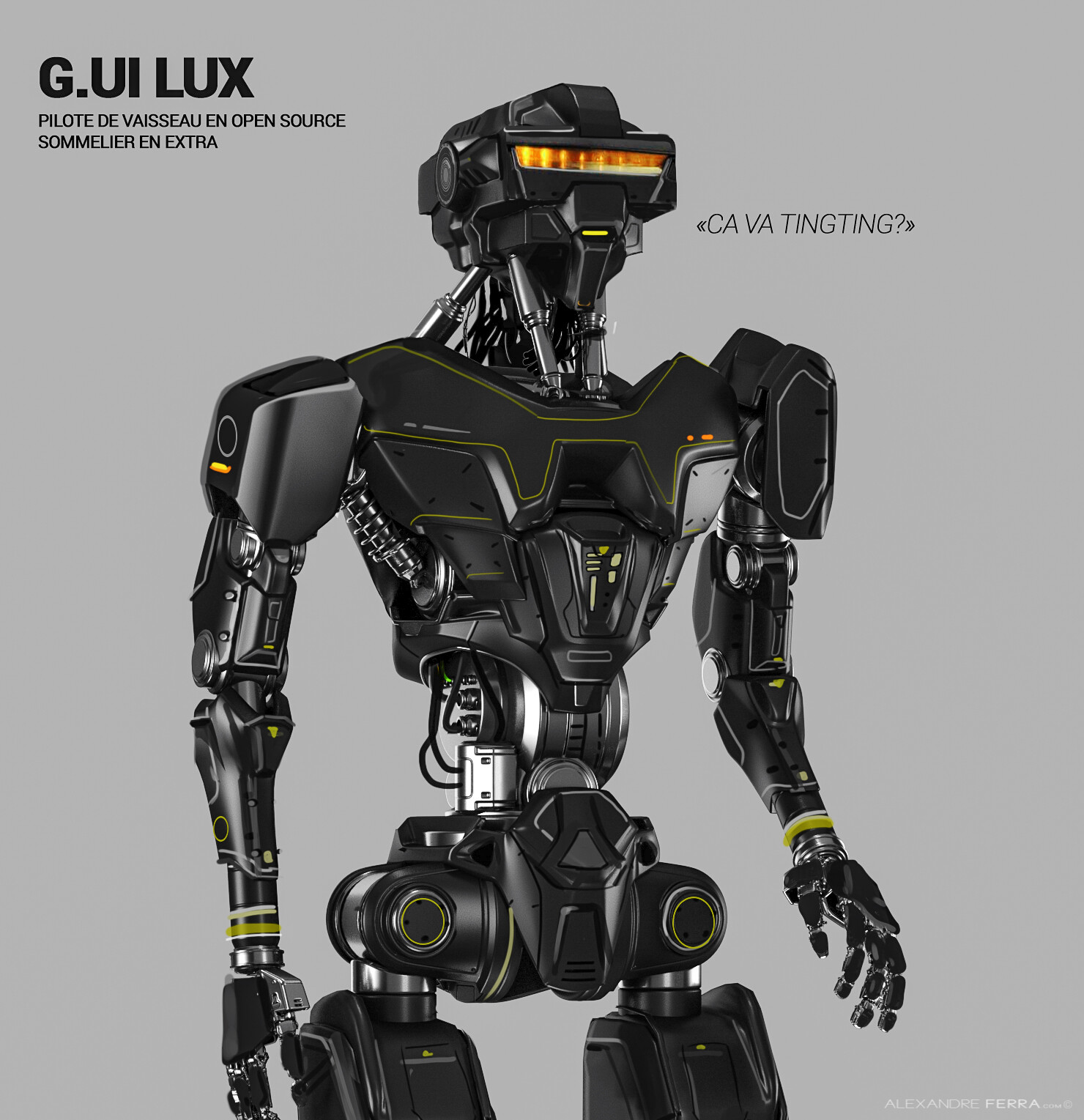This detailed photograph features a bipedal humanoid robot, primarily black with yellow and orange accents. The robot has a visor-like eyepiece reminiscent of Geordi's from Star Trek, lit with orange and yellow lights. A slit of yellow runs where the mouth would be, and you can see pipes extending from the head down to the body. Positioned against a gray background, the upper left corner of the image showcases bold text that reads "G.U.I. LUX" in black block letters, followed by smaller text: "PILOTE DE VAISSEAU EN Open Source Sommelier EN Extra." The robot's wrists and various parts of its body, including the hips, are trimmed with yellow, and it features silver components. To the right of the head, the text "CA VA TING TING?" is visible in black lettering. The bottom right of the image credits "Alexandra Ferra." The robot's design and posture suggest a mean, law enforcement appearance, potentially resembling a police bot.